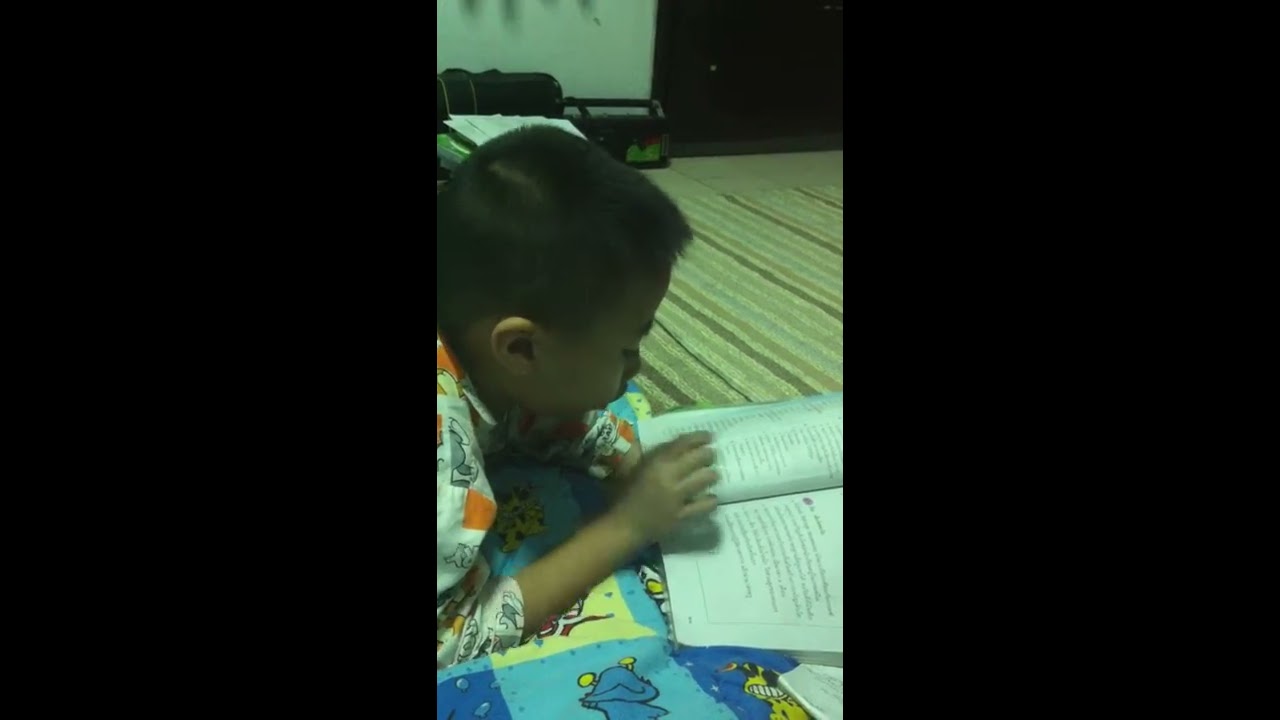In the center of the horizontally aligned rectangular image, a small boy, who appears to be between five and eight years old, is lying down on a striped area rug with brown, green, beige, and mustard stripes. The boy, with very short black hair, is visible from his shoulders up, and is shown lying on his right side, engaged with an open paperback book that has larger text, suggesting it is a child's book. His right hand is placed on the book as he reads. The boy is wearing a T-shirt with orange, white, and grey colors, and is also resting on a patterned child’s blanket adorned with a cartoon design that features a blue frog with yellow eyes or blue blobs with yellow antennae. The room's background includes part of a cream or white wall, a black sofa near the wall, and a brown door. The image is flanked by wide black vertical bars on the left and right sides, leaving only the narrow vertical center section visible.